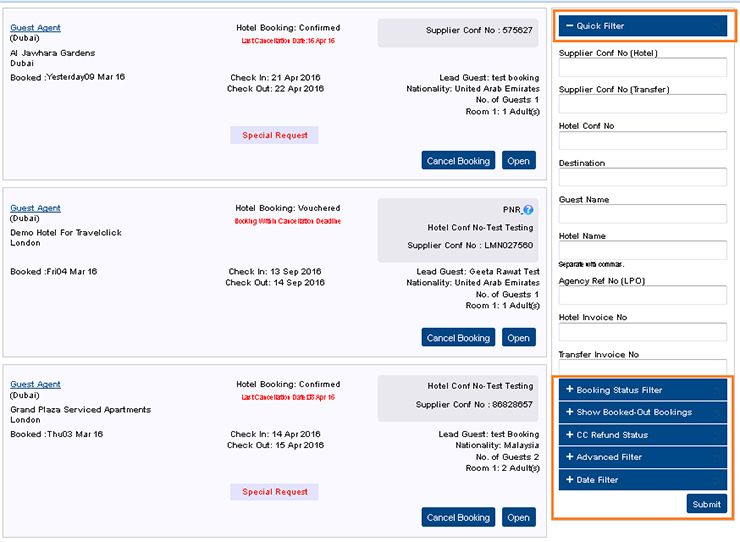**Detailed Caption:**

The image captures a detailed screenshot of multiple hotel bookings made by a guest agent in Dubai. The bookings are listed as follows:

1. **Ali Jahar Gardens, Dubai:**
   - **Date Booked:** March 10th, 2009
   - **Guest Check-in:** March 21st, 2009
   - **Guest Check-out:** March 22nd, 2009
   - **Booking Status:** Confirmed
   - **Special Request:** (Gray Box)
   - **Lead Guest:** Test Booking 
   - **Nationality:** United Arab Emirates
   - **Number of Guests:** 1 adult
   - **Room:** 1 room

2. **Dimo Hotel for Travel Click, London:**
   - **Date Booked:** March 10th (Friday)
   - **Booking Status:** Vouchered
   - **Booking Cancellation Deadline:** (Not specified)
   - **Guest Check-in:** September 13th, 2010
   - **Guest Check-out:** September 14th, 2010
   - **PNR:** (Question Mark)
   - **Hotel Conference Number:** Test Testing
   - **Lead Guest:** Greta Rantat Test 
   - **Nationality:** United Arab Emirates
   - **Number of Guests:** 1
   - **Room:** 1 room

3. **Grand Plaza Service Apartments, London:**
   - **Date Booked:** March 3rd
   - **Booking Status:** Confirmed
   - **Guest Check-in:** March 14th
   - **Guest Check-out:** March 15th
   - **Lead Guest:** Test Booking 
   - **Nationality:** Malaysia
   - **Number of Guests:** 2
   - **Room:** 1 room

The background of the screenshot is gray, and each booking entry is presented in a structured manner.